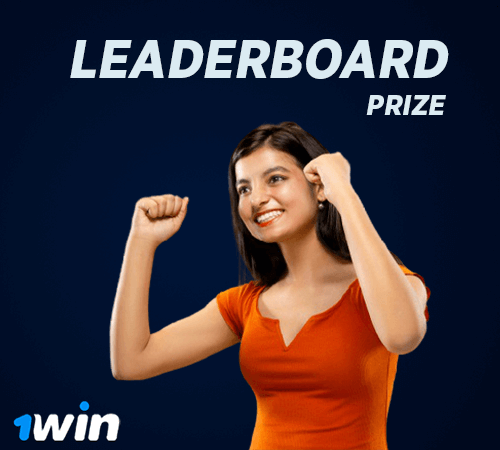The image features a young, attractive brunette woman with straight dark brown hair, smiling broadly in excitement. She's wearing an orange short-sleeved t-shirt with a V-cutout, and her arms are raised in a cheering pose, bent at the elbows. She is adorned with silver earrings and makeup, including lipstick. The background is a solid dark blue, with text at the top that reads "LEADERBOARD PRIZE" in uppercase letters, in a white or very light blue font. In the bottom left corner, the text states "one win," with the numeral "1" and the dot of the "i" in "win" highlighted in blue. This image appears to capture a moment of victory, possibly related to a competition, trivia, or gambling event.